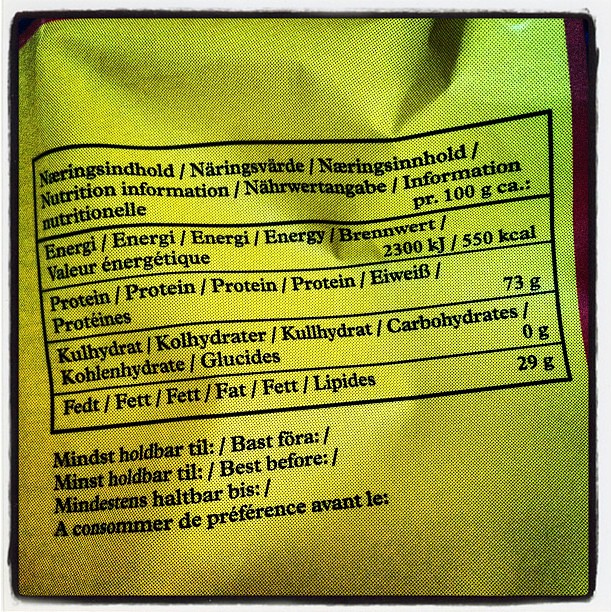This image displays a detailed nutrition label written in multiple languages. The label is divided into several sections, each denoting different nutritional components. There are five main columns, each marked with titles in various languages.

1. The first column is titled "Nutritional Information."
2. The second column lists "Energy" values, also in multiple languages.
3. The third column indicates the amount of "Protein."
4. The fourth column is dedicated to "Carbohydrates."
5. The fifth column shows the "Fat" content.

The nutritional values are given per 100 grams serving. Specifically, the label indicates that each 100 grams contains:
- 550 kilocalories
- 73 grams of protein

The label is meticulously structured to provide comprehensive information to the reader.